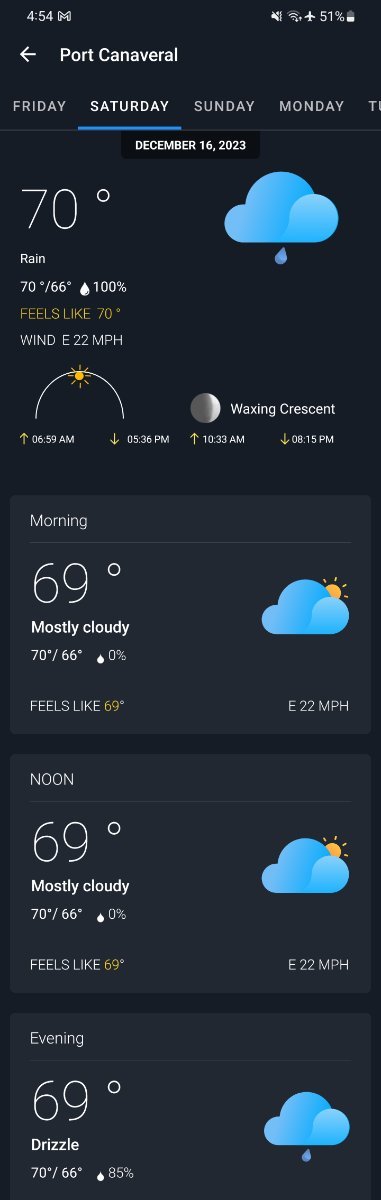This image is a detailed screenshot from a cell phone, set against a solid black background. The top part of the screenshot displays the device's status bar with white text; the current time is 4:54 AM, located at the top left. On the top right, there are indicators showing that the sound is off, the airplane mode is activated, and the battery is at 51%.

Below the status bar, bold white text provides navigation and location information: an arrow pointing left followed by "Port Canaveral." The next line displays the days of the week—Friday, Saturday, Sunday, and Monday—with "Saturday" highlighted in blue and bold, indicating the current day. Beneath it, "December 16th, 2023" is mentioned.

The weather forecast is detailed next, starting from the left:
- "70° Rain" with a high of 70°F and a low of 66°F and a rain probability of 100% indicated by a raindrop symbol.
- "Feels like 70°" is written in yellow text.
- The wind is coming from the east at 22 miles per hour.
- The sunrise is at 6:59 AM, and the sunset is at 5:36 PM, with respective icons for the sun's rise and set times.
- An image of the moon with the words "Waxing Crescent" describes the lunar phase.

Further below, additional morning weather details are provided:
- "69° Mostly Cloudy"
- High of 70°F and low of 66°F
- "Feels like 69°"

This image provides a comprehensive snapshot of the weather and essential information for Port Canaveral on December 16th, 2023.